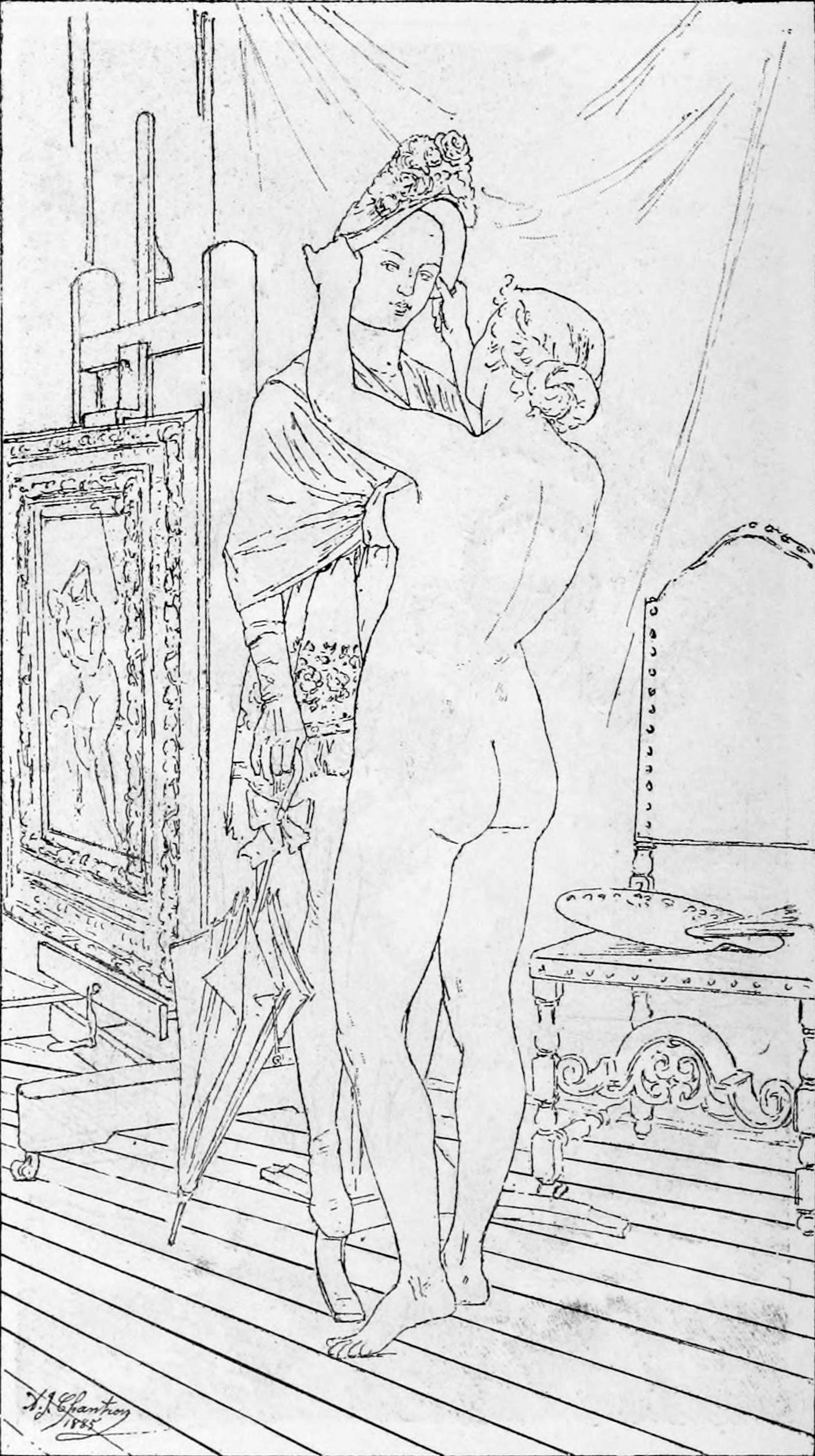This detailed black-and-white drawing, dated 1885 and possibly labeled with the initials "VJ Chantroy," depicts an intimate scene featuring two women. One woman, entirely nude with her hair tied back into a bun, stands with her back to the viewer. She is in the act of dressing the other woman, or possibly outfitting a mannequin. The nude woman is holding a wide-brimmed hat adorned with flowers, positioning it on the head of the other figure, who is partially dressed in oriental-style attire, including a short dress, a shawl draped over her shoulders, and elbow-length gloves. The dressed figure also holds a closed parasol.

The setting is a room with a wood floor composed of diagonal slats. To the right of the nude woman is a chair, atop which rests a painter's palette. In the background, a curtain or blanket hangs from the wall, and to the left, a framed portrait of a lounging nude woman on the wall further enhances the artistic atmosphere. The monochromatic color palette of the drawing emphasizes the intricate details and the interplay of light and shadow in the scene.